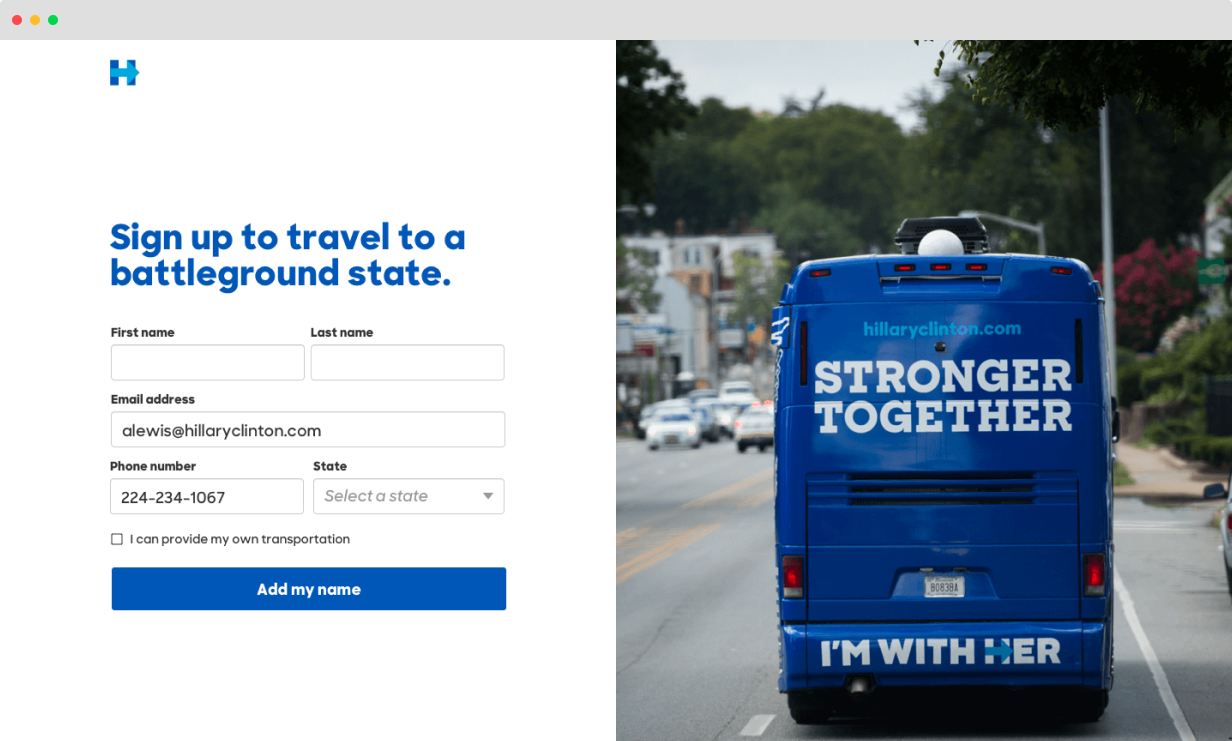The image features a recruitment advertisement urging individuals to travel to battleground states for political campaigning. 

At the top, the advertisement is adorned with green, red, and yellow circular icons, and a grey bar. In the center, there is a prominent blue "H" with a forward-pointing arrow, representing the Hillary Clinton campaign logo. Below this, the text prominently reads: "Sign up to travel to a battleground state." This call to action is repeated for emphasis.

The form fields visible in the image request various personal details: first name, last name, and email address (with an example given as always@hillaryclinton.com), along with a phone number, 224-234-1067. There is a dropdown menu option for selecting a state, though it is not selected, and a checkbox where volunteers can indicate if they can provide their own transportation.

A blue bar at the bottom invites users to "Add My Name". The background of the image shows a gray sky, green trees, and flowers, set against buildings and a gray ground. A bus, marked with distinct lines, can be seen in the center. 

The bus and the background are further branded with the slogans "Stronger Together" and "I'm With Her" adjacent to the Hillary Clinton campaign logo, featuring the recognizable blue "H" with an arrow.